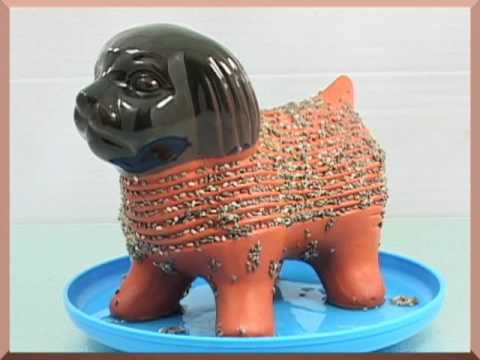This detailed photograph captures a dog-shaped Chia pet, artfully blending a black, glass-like glazed head with a reddish-brown, unglazed clay body. The dog's expressive eyes and nose add a touch of realism to its sculpted head. Its body features horizontal ridges where Chia seeds have been meticulously smeared, ready to sprout green "hair." The figure stands proudly on a blue, plastic dish, which contains a bit of water, all placed atop a white countertop against a seamless white wall. The image, taken indoors, frames the dog statuette facing towards the left, emphasizing its detailed craftsmanship and the potential for verdant growth.